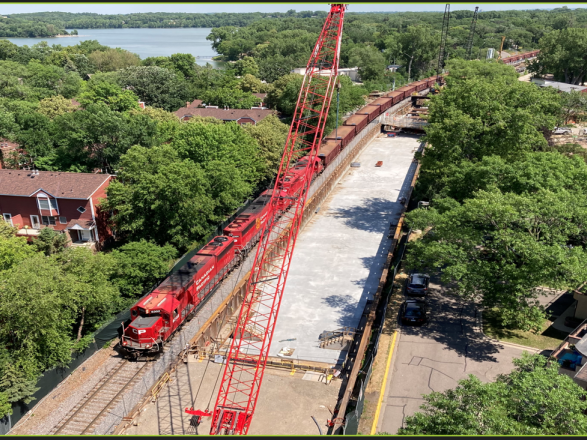This aerial photo captures a vibrant red train curving gently from the bottom left to the top right of the image along a winding train track. The train comprises an engine car followed by two more red cars, and a series of brown freight cars carrying several large brown, rectangular cargoes. The scene is set amidst a lush green landscape filled with tall, bushy trees and brown houses nestled into the forested area, adding a quaint residential touch. In the foreground, to the right of the train track, a red construction crane stands prominently, its color echoing the hue of the train. This crane appears to be part of a construction project running parallel to the tracks. In the distance, a serene body of water, likely a lake or river, shimmers in the sunlight. A sliver of blue sky at the very top of the image completes this picturesque scene.